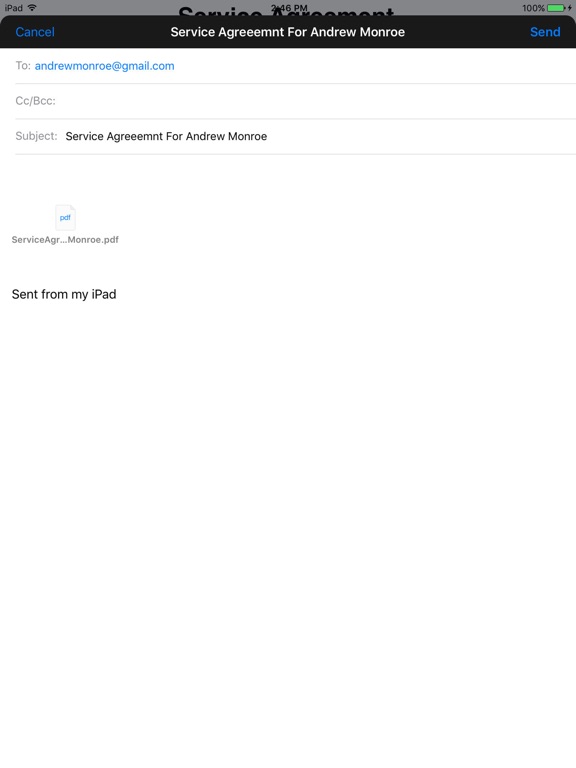Detailed Caption: 

The image depicts a service agreement page displayed on an iPad. At the very top, a light gray rectangle spans from left to right, featuring several elements: on the upper left corner, the word "iPad" appears in black text, followed by a Wi-Fi signal indicator. Centered within this rectangle is the text "Service Agreement" in black, with the time "3:16 PM" positioned directly above it. To the far right, "100%" is displayed in black text next to a green battery indicator.

Below this, a darker black rectangle also extends from left to right, with its top corners rounded. On the left side of this rectangle, the word "Cancel" appears in blue text. In the center, the text "Service Agreement for Andrew Monroe" is prominently displayed in white. On the far right of the rectangle, "Send" is shown in blue text.

Following this black rectangle, the document details are listed as follows: the line labeled "To" is followed by "andrewmonroe@gmail.com" in blue text. Below this line, a light gray separator runs from left to right. Beneath it, the text "CC/BCC" is displayed, followed by another light gray separator.

Further down, the section labeled "Subject" contains the text "Service Agreement for Andrew Monroe." This is also followed by a light gray line extending horizontally. Below the subject line, there is an icon representing a PDF document titled "service_agreement_Monroe.pdf."

At the very bottom, the phrase "Sent from my iPad" is displayed in the same black text.